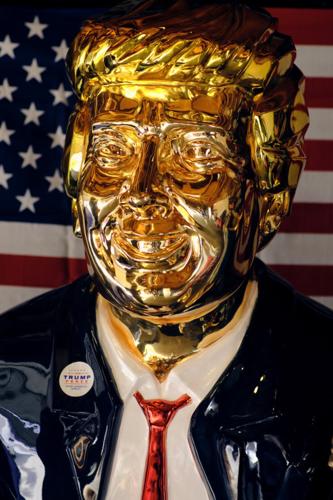This photograph depicts a statue of Donald Trump, showcasing his head and upper body. The statue's head and hair are made of a shiny, gold-painted material that resembles the look of C-3PO from Star Wars, although it appears somewhat crudely rendered. The exaggerated features give it a grotesque appearance. The figure is adorned in a navy blue coat, a white collared button-down shirt, and a red tie. Prominently displayed on his right lapel is a mostly white, circular political button inscribed with the name "Trump" and additional text. The backdrop of the photograph features a partially visible American flag, displaying both blue with white stars and red and white stripes. The image is taken in portrait orientation, capturing the reflective qualities of the statue's gold surface and the texture of its attire, contributing to the overall striking and somewhat surreal appearance.